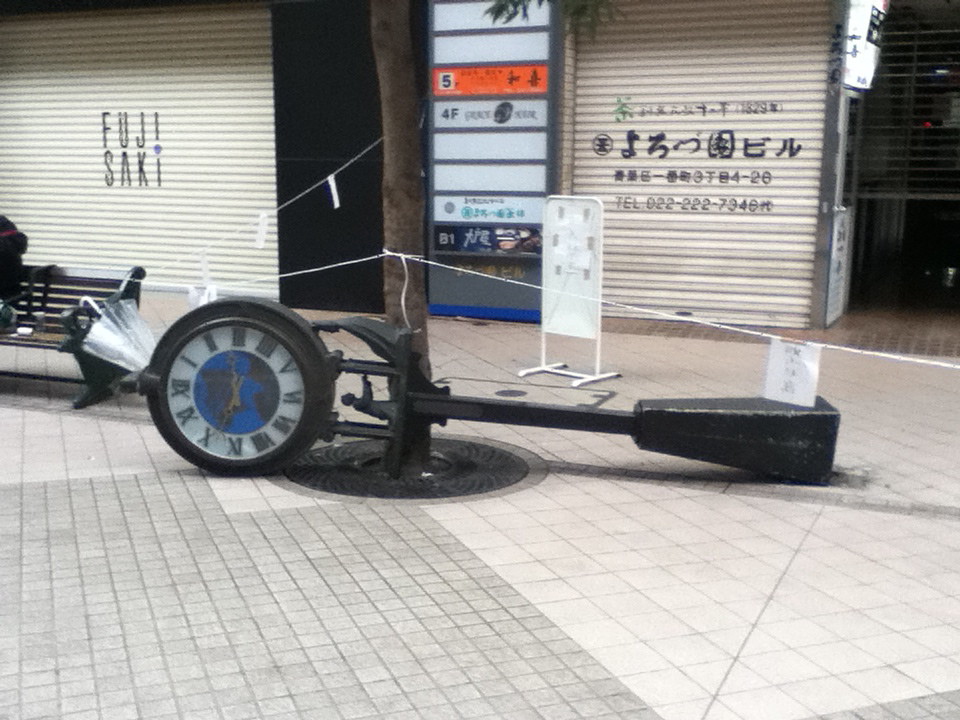The image captures an outdoor area bustling with shops, characterized by a fallen clock on a pole that lies on its side. The clock pole, made of black metal, features an obelisk-shaped base. The top of the pole has a detailed design, emphasizing a sculpted human figure between two small pillars. Encased in a black rim, the clock itself displays Roman numerals and houses a blue and green globe at its center.

The scene is set on a checkered street paved with beige tiles. Behind the central fallen clock, various shops are visible in close-up. One of the shops has a prominent white sign with the word "Fujisaki." To the upper right, signs adorned with Asian characters are noticeable. Additionally, a display board stands out with strips of different colors, including predominantly white, one orange strip, and one black strip, listing various businesses in the vicinity.